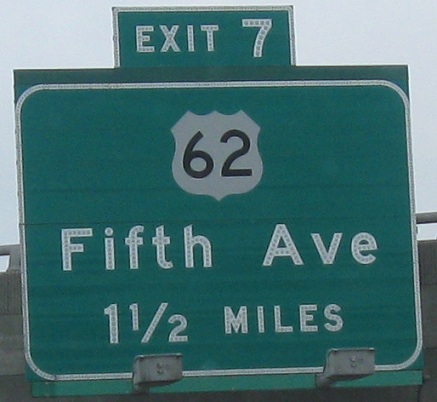The image depicts a large green highway exit sign for "Exit 7" which directs drivers towards Route 62 and 5th Avenue, 1.5 miles away. The sign is prominently mounted on an overpass and clamped securely to its structure, with the overpass running horizontally across the scene. The background of the sign is accentuated with a black border, and it is flanked by two metal lights designed to illuminate it during nighttime. If you were driving, you would encounter this sign as you approach and travel underneath the overpass, ensuring clear visibility for all commuters.